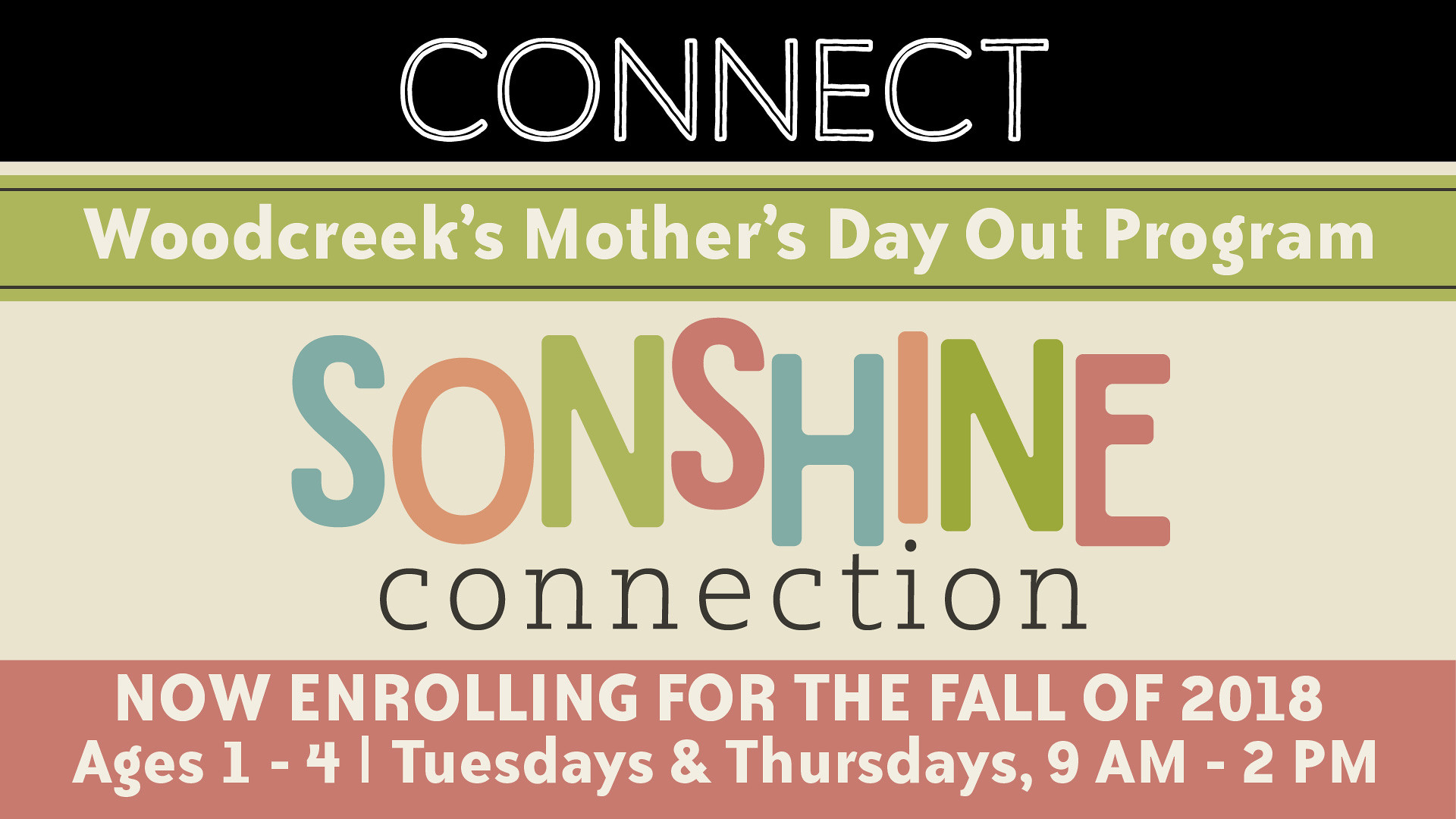The image is a promotional poster for Woodcreek's Mother's Day Out Program, titled "Connect," and prominently features the tagline "Sunshine Connection" (stylized as "Son-Shine Connection"). The poster announces enrollment for the fall of 2018, stating that the program is available for children ages 1 to 4 and operates on Tuesdays and Thursdays from 9 a.m. to 2 p.m. The design elements include a green background with the word "Sunshine" displaying in a spectrum of colors, each letter varying in hue. The poster occupies the entire image, with no other objects present. The overall aesthetic suggests a vibrant and engaging advertisement aimed at parents looking for early childhood education or childcare options.